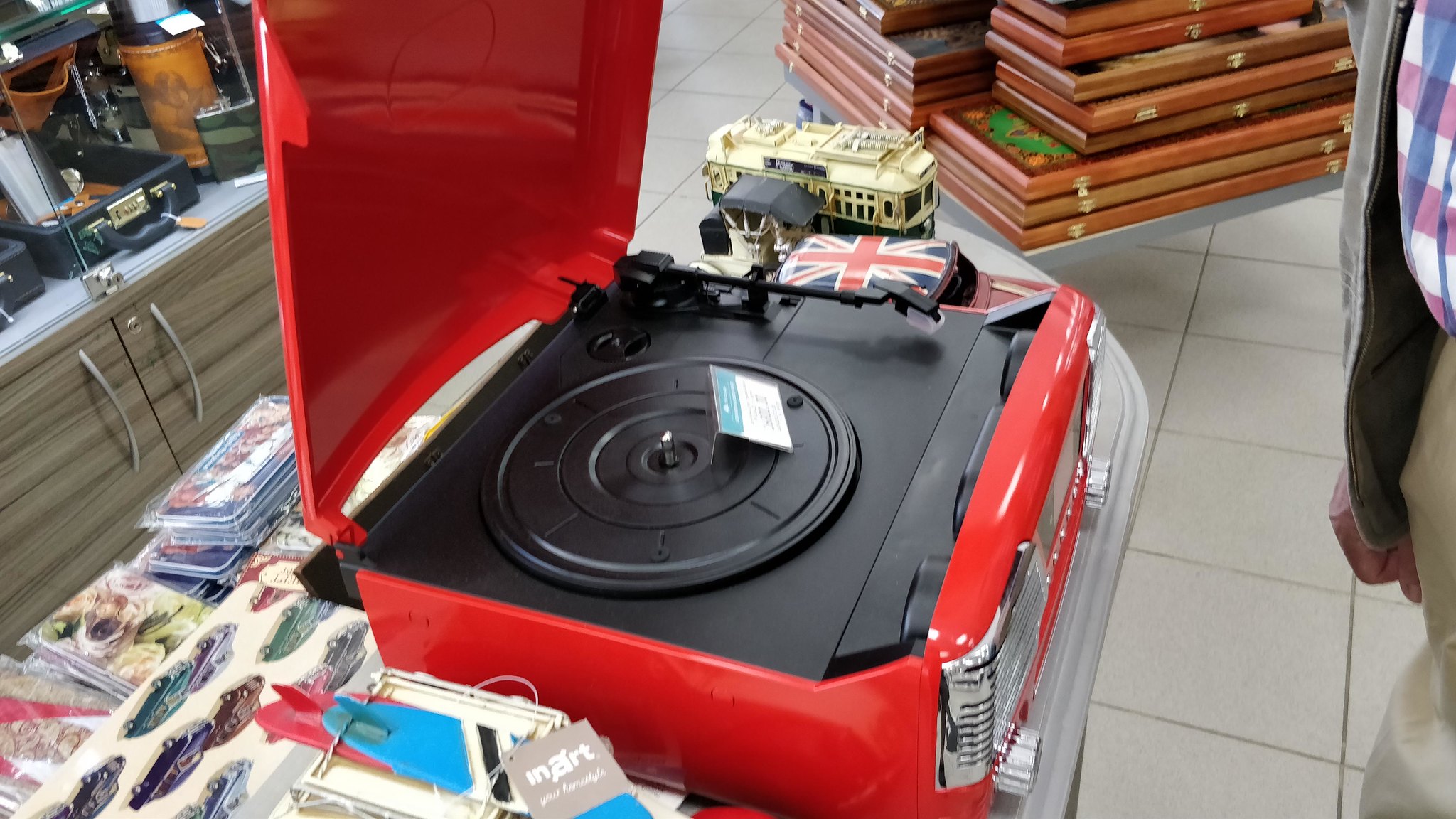This photograph features a vibrant display centered around a red retro-themed vinyl turntable styled to resemble the boot of a car, complete with a silver grill, knobs, and dials on the front. The turntable, with a sleek black interior, is positioned prominently on an island bench amidst various nostalgic items available for sale. These items include small model cars, stickers of classic vehicles, a Union Jack-patterned Mini Cooper model, and other vintage memorabilia. To the left of the turntable, an array of items such as surfboards and a small model building is visible. Additionally, a briefcase filled with undisclosed items and a locked glass cabinet adds to the eclectic assortment in the background. Also noticeable are timber-framed pictures and a model tram on display. A partially visible person stands on the right side of the image, observing the setting. This scene, likely set in a thrift store or antique shop, is characterized by its warm, nostalgic ambiance accentuated by brown hues and detailed wooden decor.